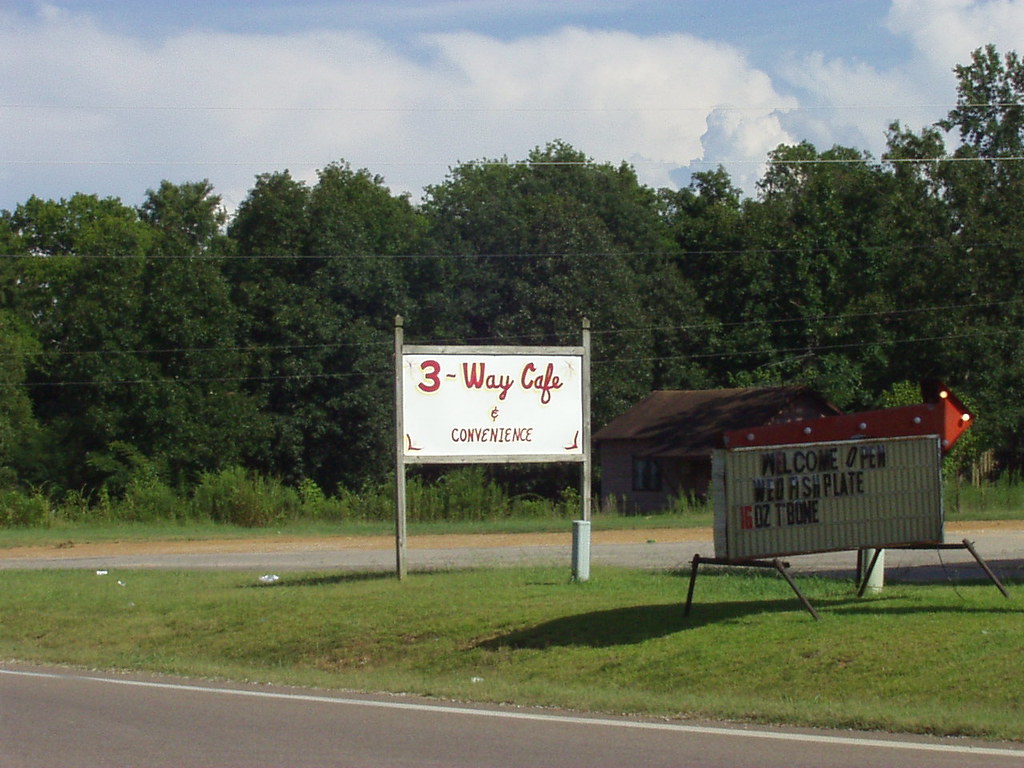The image showcases a vibrant outdoor scene featuring a wooden signboard and a smaller billboard positioned on the ground in front of a store. The wooden sign prominently displays the name "Three-Way Cafe and Convenience." The accompanying ground-level billboard boasts a welcoming message: "Welcome Open. Red Ash Plate 16 ounces T-bone," accompanied by a striking red arrow pointing to the right. The arrow is adorned with several lights, only two of which are illuminated, possibly due to the daylight conditions. The background reveals a serene setting with numerous trees and a quaint house, enhancing the quaint and inviting atmosphere of the locale. The overall quality of the image suggests it was likely taken with an older digital camera, contributing to the scene's nostalgic and vibrant charm.